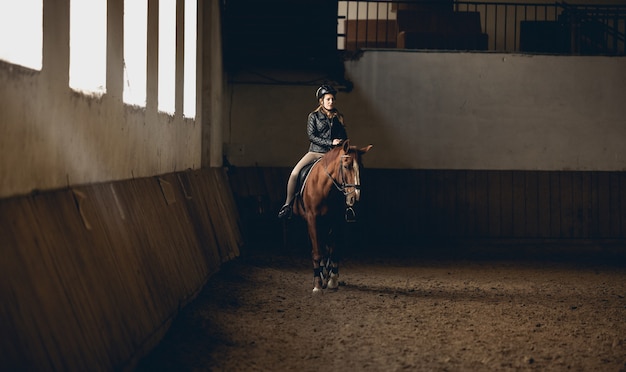In this detailed photograph, a white woman with long brown hair, wearing a black helmet, black riding jacket, and riding pants, is seen atop a robust, dark brown horse with noticeable white markings on its nose and hooves. The horse, equipped with reins, stands solemnly on a sandy ground within what appears to be an indoor riding arena or barn. The scene is bathed in natural light streaming through five windows on the left wall, casting shadows on the right side of the arena. The surroundings include protective wooden planks at the bottom of the walls and clay elements above them. In the background, there's a railing that appears to lead to a viewing area or possibly a second story, enhancing the arena's structured environment. No other people or animals are present in the image.